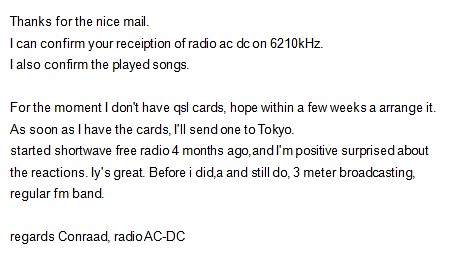The image features a white background with centrally positioned, black typed text resembling an email or letter from a radio station named Radio ACDC. The content of the text reads: "Thanks for the nice mail. I can confirm your reception of Radio ACDC on 6210 kHz. I can confirm the played songs. For the moment, I don't have QSL cards. I hope to arrange it within a few weeks. As soon as I have the cards, I'll send one to Tokyo. Started shortwave free radio four months ago and I'm positively surprised about the reactions. LY is great. Before I did and still do 3-meter broadcasting on the regular FM band. Regards, Conrad, Radio ACDC." The message is split into two paragraphs followed by the closing remarks and is set in a standard type font.